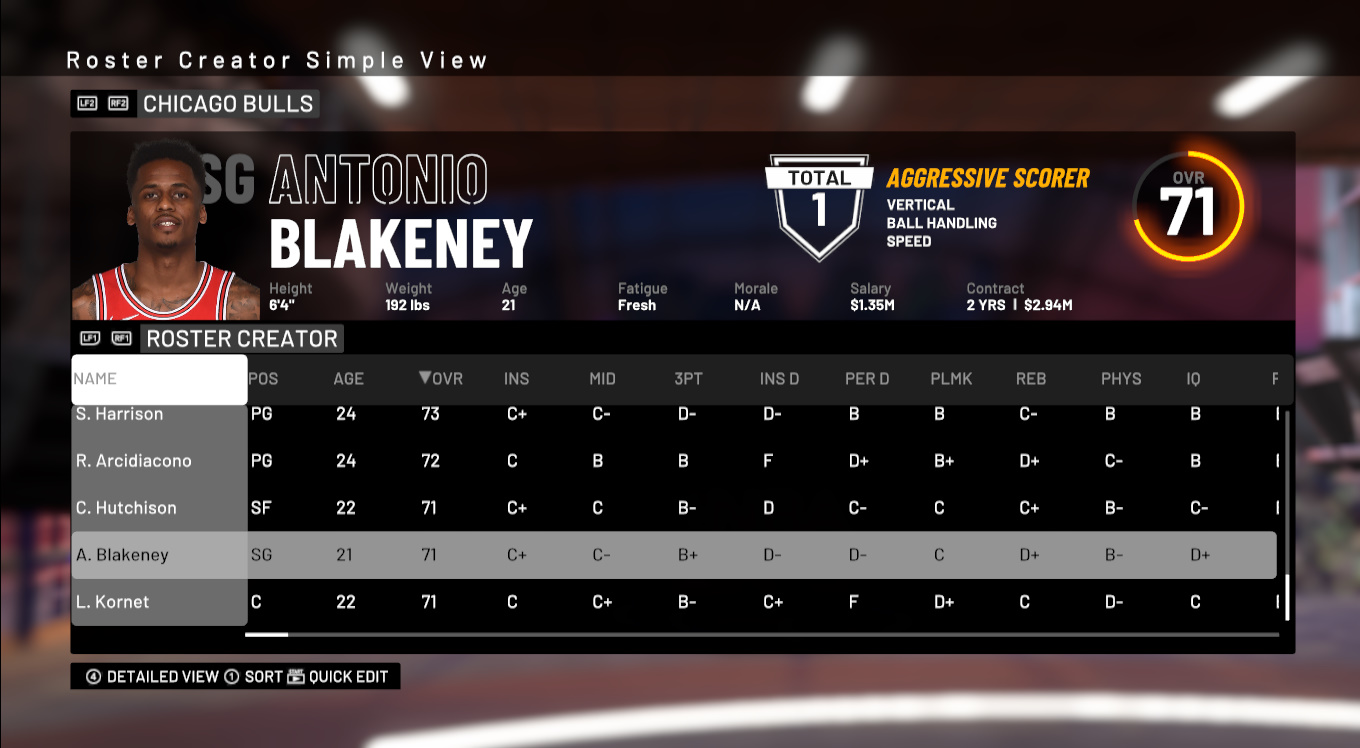In the image, the top right corner displays the text "Roster Creator: Simple View." Below that, the text reads "Chicago Bulls" and "SG Antonio Blakeney." There's a picture of Antonio Blakeney wearing a basketball jersey. His details are written as follows: height is 6'4", weight is 192 lbs, age is 21, fatigue level is fresh, morale is N/A, salary is $1.35 million, and contract is 2 years for $2.94 million.

Above these details, it mentions "Total: 1 Aggressive Scorer" with attributes such as vertical, ball handling, and speed. His overall rating is 71, indicated by orange text that's nearly full. On the left side, beneath the username, the text "Roster Creator" appears again, followed by names with their respective details: S. Harrison, R. Arcidiacono, C. Hutchison, A. Blakeney (highlighted as selected), and L. Kornet.

In the bottom left corner, there is text indicating "Detail View," "One Shot," and "Quick Edit." A table lists detailed stats for S. Blakeney, position SG: age 21, overall 71, with performance grades - inside: D-, perimeter defense: D-, playmaking: C, rebounding: D+, athleticism: B-, basketball IQ: D+. The table also includes stats for other players: S. Harrison (age 24, overall 73), R. Arcidiacono (age 24, overall 72), C. Hutchison (age 22, overall 71), and L. Kornet (age 22, overall 71).